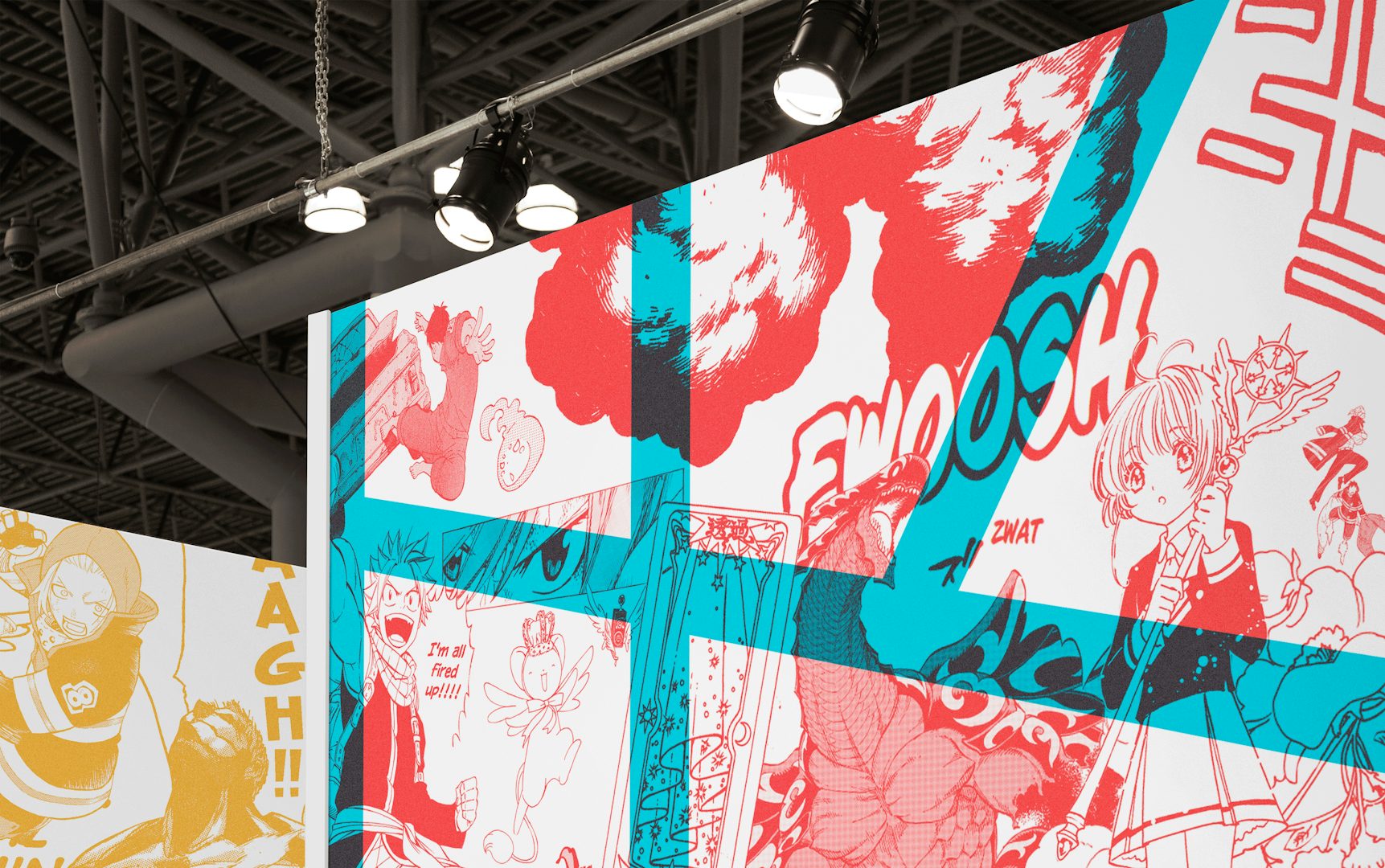The image depicts an indoor scene at what appears to be a convention center or conference venue, characterized by a high, gray ceiling adorned with visible rails, vents, piping, and brightly lit hanging lights. Central to the image are temporary display walls or boards designed to resemble comic book pages, covered with colorful anime-style artwork and text. The displays feature a vibrant array of characters and scenes: a girl holding a scepter or stick with wings and a star at the end, a nearby dragon, a boy with spiky hair exclaiming "I'm all fired up," and various cutesy fairy creatures and animals such as monkeys. The visual composition employs a vivid palette of red, white, blue, gold, and yellow, with dynamic elements like clouds and explosions, and action words such as "ARG," "ZWAT," and "WUSH," capturing the energetic and whimsical essence of the artwork.